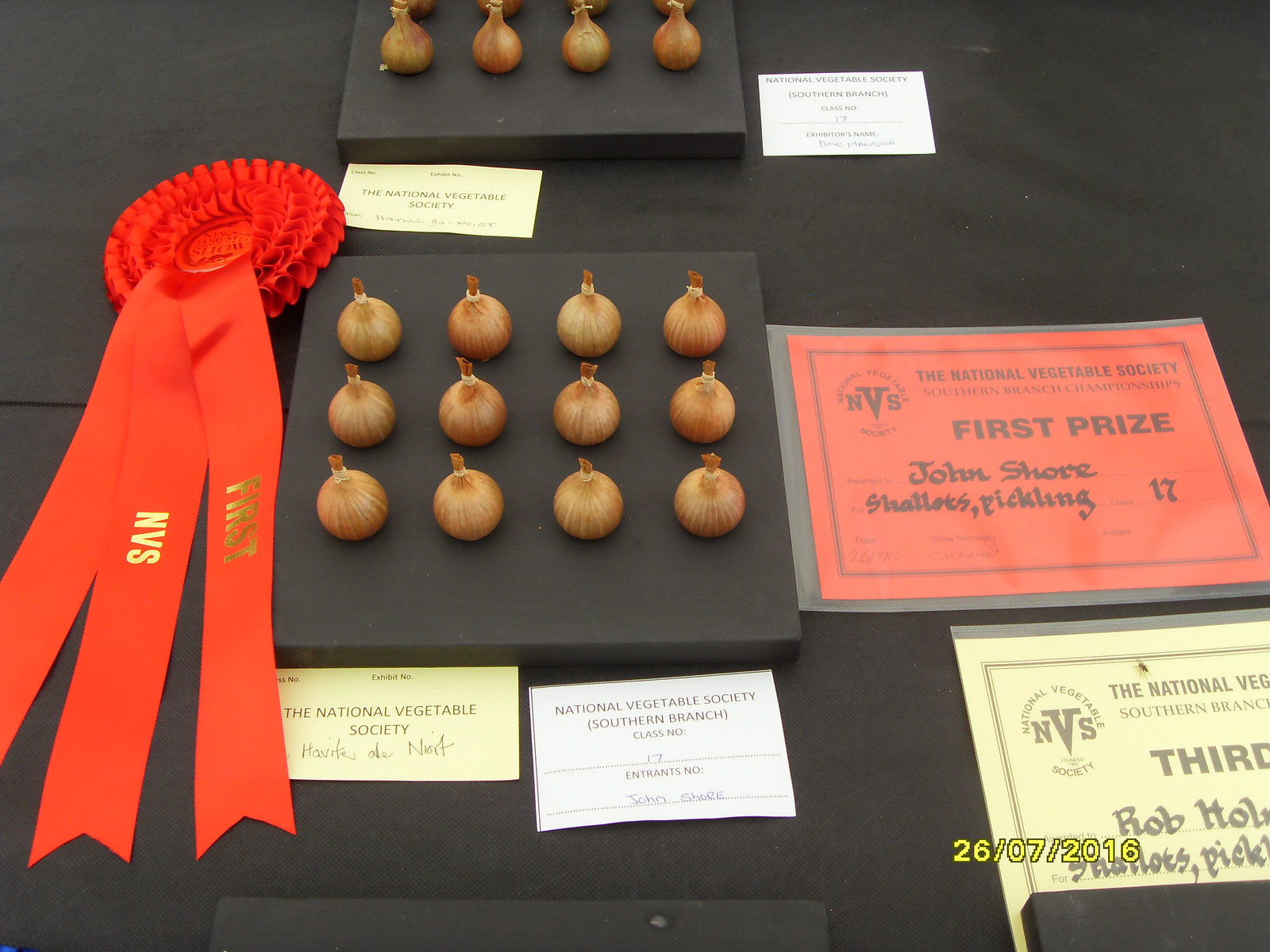In the image, we observe an award competition display of onions, specifically shallots, arranged meticulously on a black table draped with a black cloth. On the table, the shallots are displayed on square boards, organized neatly in three rows of four, totaling twelve shallots. The shallots themselves are a distinctive purple color, and their arrangement forms a neat rectangular pattern on the black stand. To the left of this display, a red ribbon with the text "First NVS" indicates a first prize win. Adjacent to this, on the right side, a larger red sign reads, "The National Vegetable Society First Prize, John Shore, Shallots Pickling, 17." The image also captures a third-place certificate with some text that is partially cut off, showing "Rob Hole" and featuring a tan green color. Decorative little cards from the National Vegetable Society are also scattered around the display, highlighting the importance of the event. In the lower right-hand corner of the image, a timestamp indicates the date "26/07/2016." This detailed presentation emphasizes the careful preparation and recognition given to the shallots in this competitive setup.